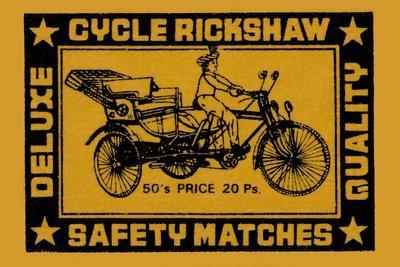The image depicts a rectangular label on a pack of safety matches, featuring a mustard-colored background framed by a thick black border. At the top, the text "Cycle Rickshaw" is cut out to reveal the mustard color underneath. Within the black frame, in each corner, there is a yellow star. On the right side, the word "Quality" is written vertically, and on the left side, "Deluxe" is also inscribed vertically. At the bottom of the frame, the words "Safety Matches" are prominently displayed. The central illustration is a pencil drawing of a cycle rickshaw: a bicycle with three wheels, piloted by a man, though the carriage seat remains empty. Below the illustration, the text reads, "50's Price 20 P.S." This detailed label emphasizes the product's attributes and includes a unique drawing that adds a vintage charm to the design.